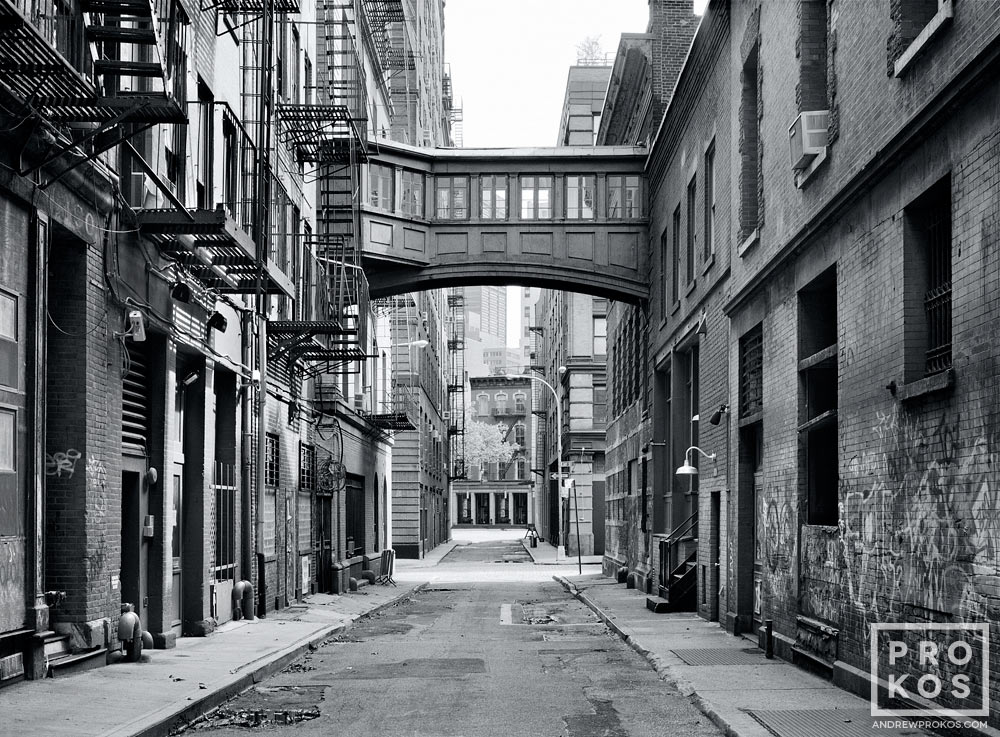This black and white photo captures a narrow cobblestone street flanked by a mix of worn-down buildings reminiscent of 1920s architecture. The scene is bathed in bright daylight, highlighting the urban grit and texture. To the left, taller buildings rise five to six stories high, complete with balconies and zigzagging fire escapes. On the right, a two-story building with windows hosts an air conditioner jutting out. A striking feature is the enclosed sky bridge adorned with windows and panels, connecting two of these historical structures mid-way up. Graffiti and street art adorn the walls, adding splashes of creative expression to the aged facades. An overhead lamp marks a doorway, while at the far end of the street, the road meets a cross-street, suggesting the urban sprawl continues beyond. Just above this junction, skyscrapers faintly mark the skyline, blending the historical with the modern. In the lower right corner, a bordered white sign reads "PROKOS," supporting the notion of timeworn resilience and artistic revival in an ever-evolving cityscape.